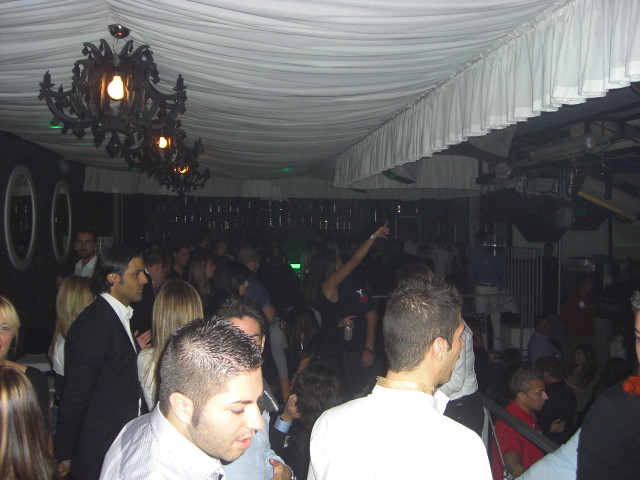This color photograph captures a lively and crowded reception event taking place inside an elegant venue. The room is adorned with white draped fabric on the ceiling, creating a tent-like atmosphere. Ornate chandeliers hang in a row, providing soft lighting that enhances the festive ambiance. The crowd, dressed in semi-formal attire, includes men in black suits, dress shirts, and collared shirts, as well as women in nice dresses. The diverse group of attendees are engaged in conversations and appear to be enjoying the occasion, holding drinks as they mill around the room. In the background, there's a bar with rows of drinks on the shelves, adding to the celebratory feel. To the right, there seems to be a stage, possibly for a band providing live entertainment, as guests are collectively facing in that direction. Two distinct features that stand out are the exit sign with a green light and the carefully arranged cabinet lights in the distance, further indicating the well-appointed nature of the venue.